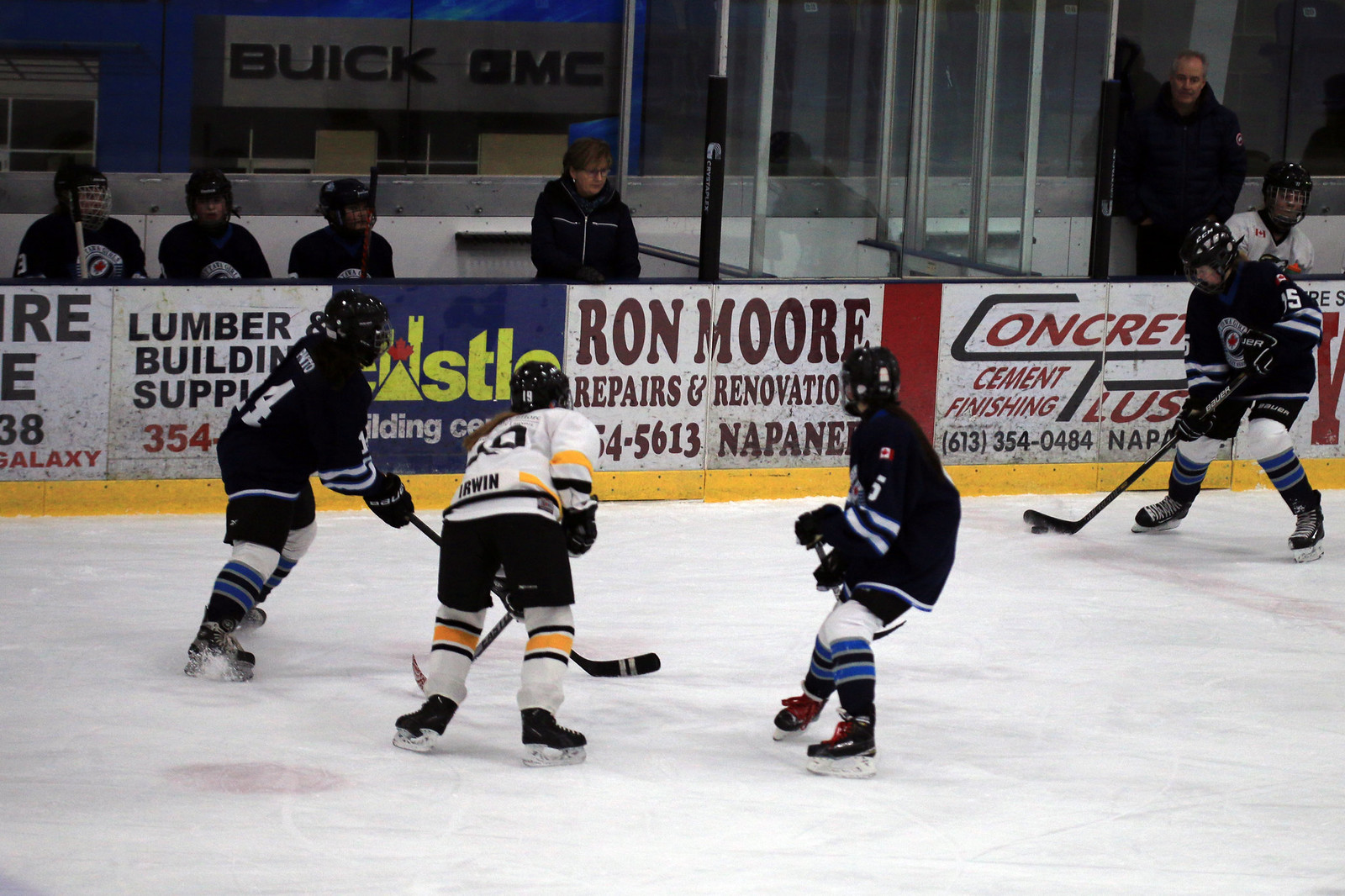The image captures a dynamic ice hockey game inside a rink lined with various advertisements. Four players are on the ice: three donning black jerseys with red pants and blue-trimmed socks, and one in a white jersey with black pants and gold trim. The action centers on a player at the far right, poised to strike the puck, while the others focus intently on the play. Surrounding the rink, a barrier showcases an array of ads. From left to right: a partially obscured black-text ad likely reading "Lumber Building Supplies," a prominent brown-text ad for "Ron Moore Repairs and Renovations, 4-5613 Napani," and another ad for "Concrete Cement Finishing," followed by a blue sign showing only four yellow letters. The barrier separates the rink from the audience, with four spectators in view, and a man who appears to be in the penalty box dressed in the white team's uniform. The ice surface, slightly tilted upwards to the right, displays faint red paint markings, enhancing the scene's authenticity and competitive ambiance.